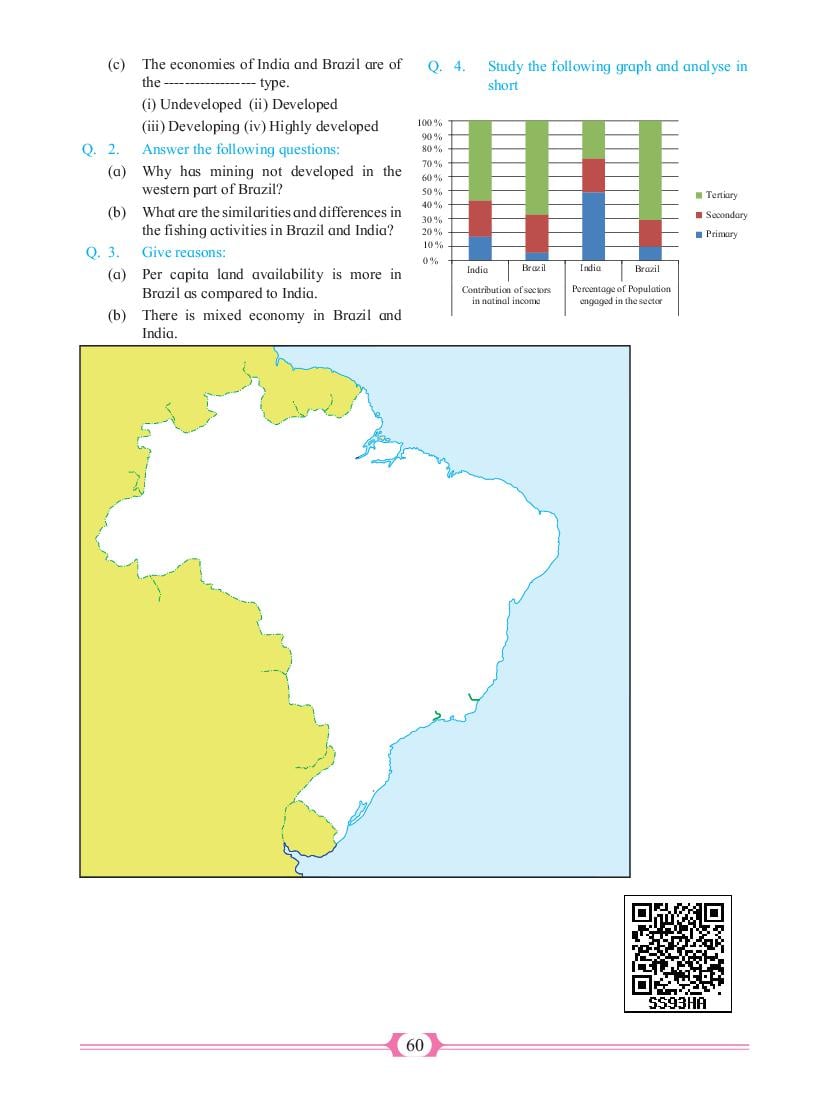The image depicts a detailed map in a mixed style, showcasing two distinct landmasses differentiated by color schemes. One landmass is marked in yellow, outlined by a blue border, while the other landmass is depicted in white, also bordered in blue. Surrounding these landmasses is a sky blue area, symbolizing water. In the bottom right corner, there is a QR code labeled "SS93HA." A pink-bordered section at the bottom features the number "60," likely indicating a page number from a book where the image originated.

At the top of the image, there are several questions and answers focused on the economies and geographic characteristics of India and Brazil. The first question provides multiple-choice options regarding the developmental status of India and Brazil: undeveloped, developed, developing, or highly developed. Further questions ask about the reasons behind the underdevelopment of mining in western Brazil, similarities and differences in the fishing industries of Brazil and India, and the reasons behind the higher per capita land availability in Brazil compared to India. Additionally, it addresses the presence of a mixed economy in both countries.

There is also a graph for analysis, illustrating data in percentages from 0% to 100% in 10% increments. The graph includes four columns: "India for Contribution of Sectors in Nominal Income," "Brazil for Contribution of Sectors in Nominal Income," "India Percentage of Population Engaged in Sectors," and "Brazil Percentage of Population Engaged in Sectors." Each column is divided into green (tertiary sector), red (secondary sector), and blue (primary sector) segments, representing the respective contributions and population engagements in these sectors.